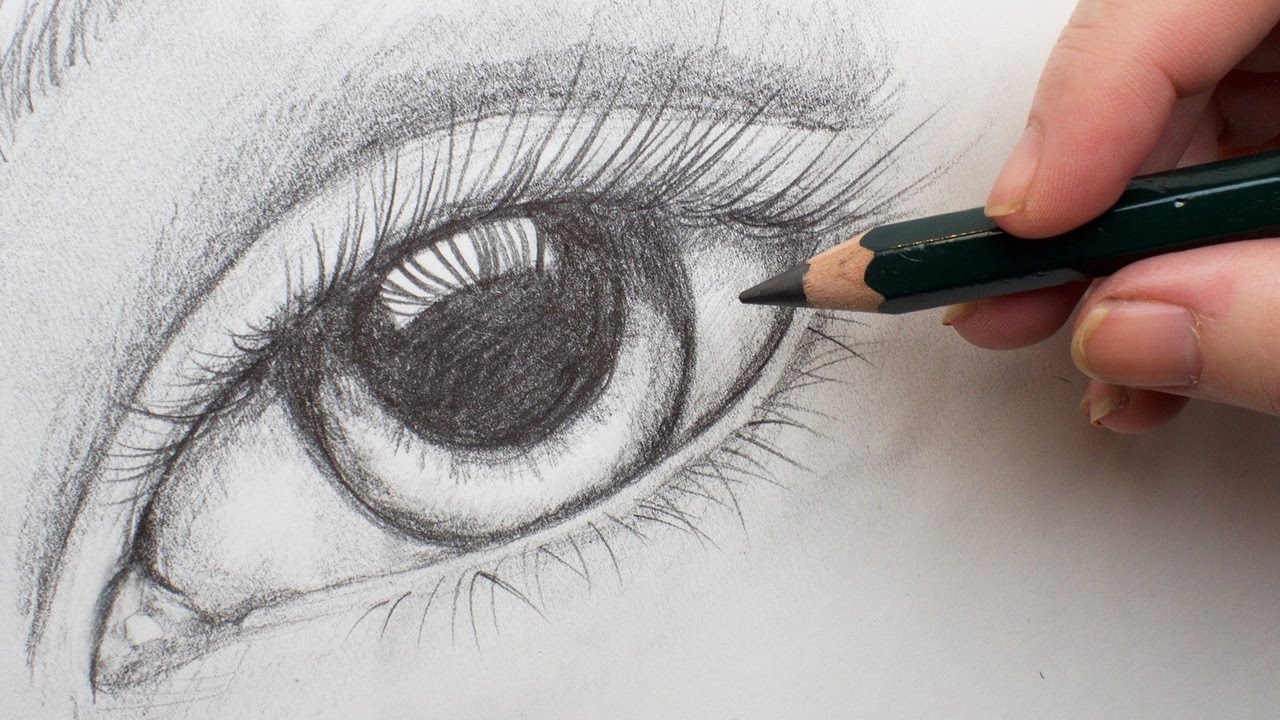In the image, a white hand with long, dirty fingernails emerges from the top right corner, holding a well-sharpened black pencil with a slightly blunt tip. The hand is actively engaged in drawing an eye on a piece of white paper, which lies beneath it. The eye, meticulously sketched, features long upper eyelashes and a detailed pupil with a distinct white reflection, lending it a lifelike quality. The iris and the surrounding areas are finely shaded, creating depth and realism. Part of the eyebrow is also visible, adding to the intricate details of the artwork in progress. The shadow of the hand is cast on the paper, enhancing the dimensionality of the scene.